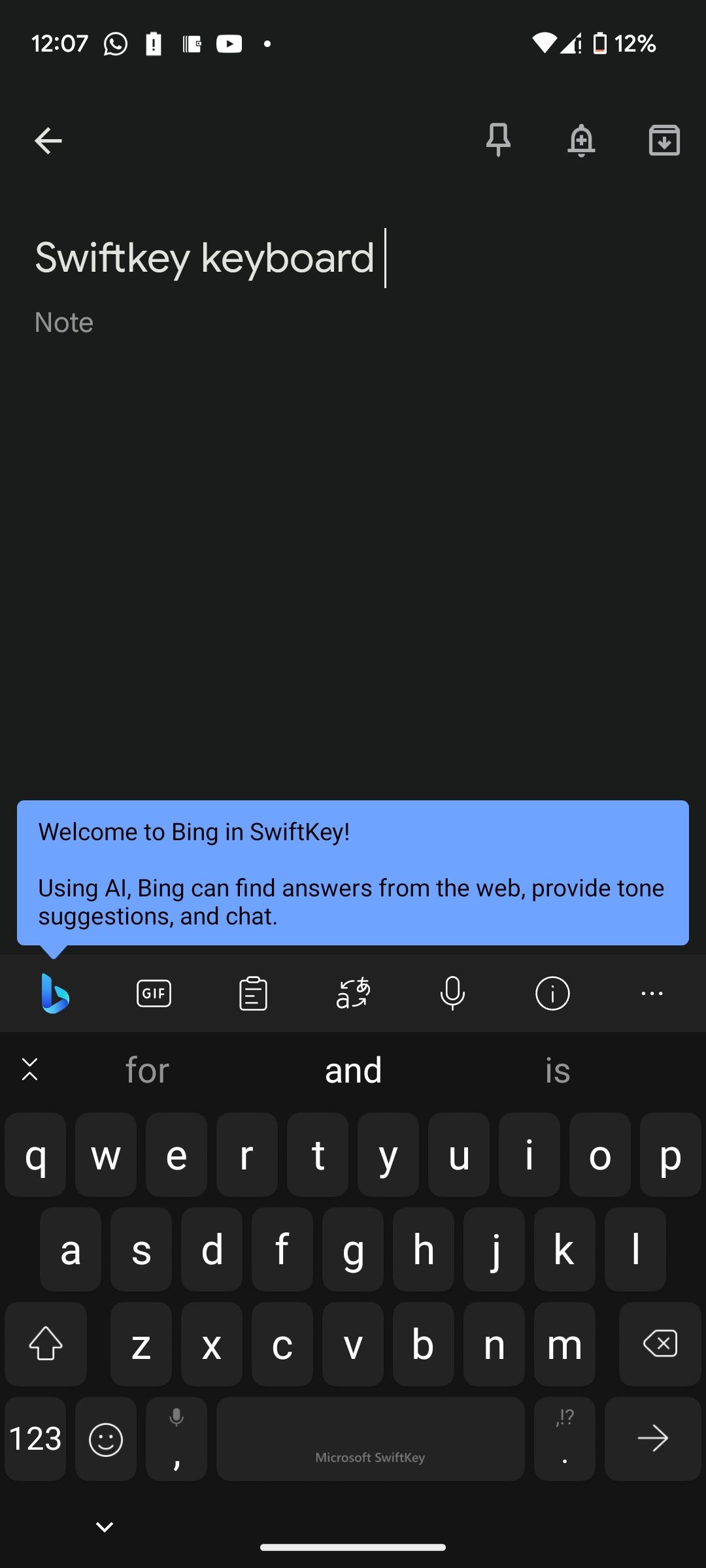Screenshot Description:

The image is a screenshot taken on a smartphone. In the upper left-hand corner, the time is displayed in white text as 12:07. To the right of the time, icons for a phone (in a speech bubble), battery, YouTube, Wi-Fi, and cellular signal are present, with the battery indicating a charge of 12%. Below these icons, a navigation bar displays a left-pointing arrow on the left side and icons for a thumbtack, bell, and a square with a downward-pointing arrow on the right. Underneath this bar, the white text "SwiftKey keyboard" is visible, followed by a vertical line.

Beneath the "SwiftKey keyboard" text, the word "note" appears in gray. Dominating the bottom part of the screen is a blue rectangular speech bubble spanning the screen's width, centered with the message: "Welcome to Bing in SwiftKey. Using AI, Bing can find answers from the web, provide tone suggestions, and chat." Finally, the cell phone's keyboard is visible at the very bottom of the screen.